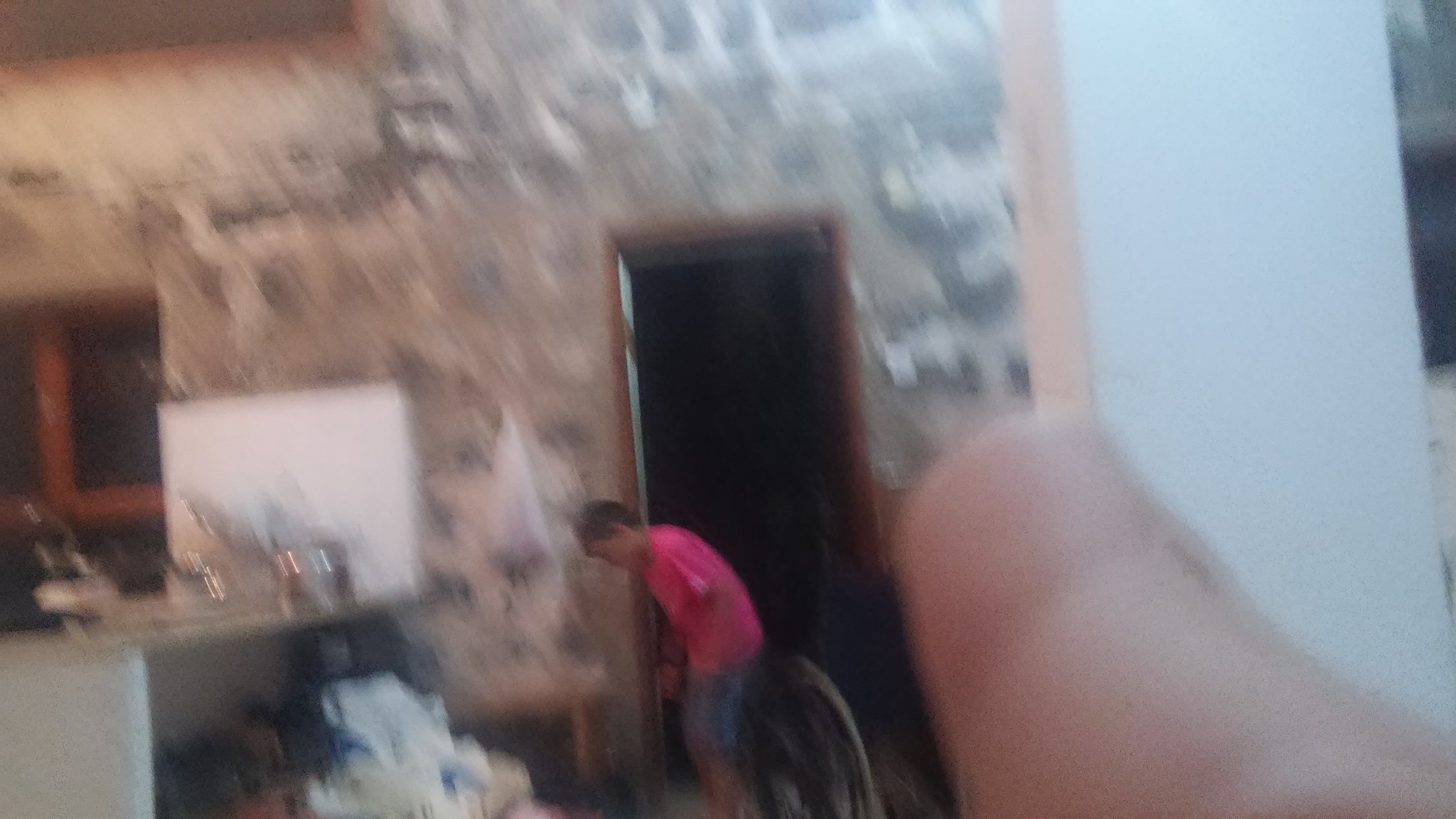The image is slightly blurry, capturing a scene that appears to be indoors. At the center, a short person with a hunched posture bent at a 40-degree angle is visible. Their knees are slightly bent, with the right arm extended in front of their knees and the left arm at knee level. The individual has short black to gray hair and a brown complexion, and is dressed in a pink short-sleeve shirt with blue shorts, revealing their legs up to the ankles, where the feet are not visible.

They stand in front of an open brown doorway, leading into a dark room. The wall around the doorway is gray and looks unfinished. To the person's left, there is a countertop with a marble top and a white base, cluttered with numerous objects. Below the countertop, various items in white, black, and blue can be seen. 

A window with brown trimming appears on the left side of the image, showing the darkness outside. On the right side, a white column occupies about a fourth of the image, with a brown object in front that seems to be a person's finger. Additionally, a plastic bag hangs on the wall to the left of the doorway.